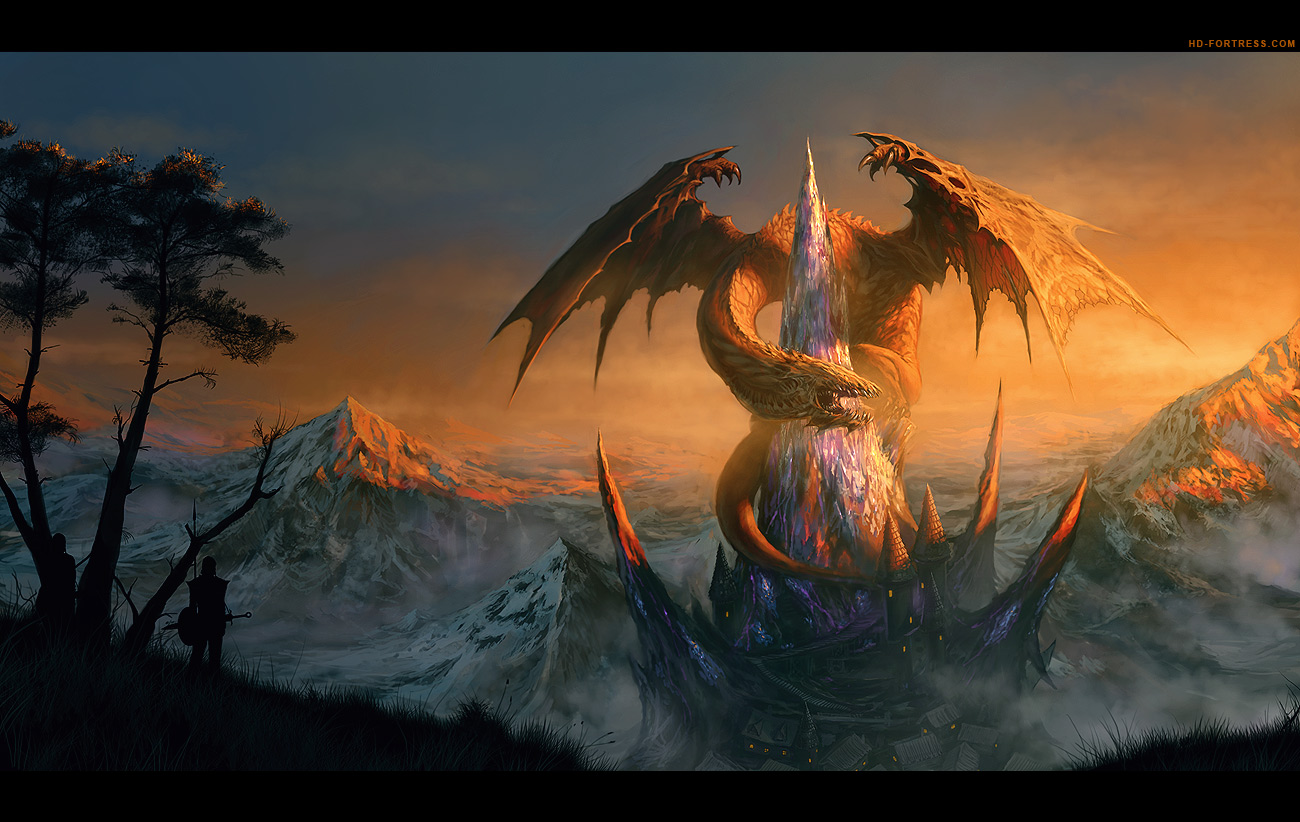The image is a detailed and dramatic digital painting that captures a fantasy scene seemingly inspired by a movie animation. It features a wide, rectangular composition with a black border on the top and bottom. The top border has the text "HDfortress.com" in an orange color on the right side. The scene itself unfolds against a dynamic, shadowy landscape with a horizon visible in places. 

On the left side of the image, there's a silhouetted tree beneath which stands a shadowy figure holding what appears to be a guitar. Central to the scene is a towering, sharp mountain peak, slightly offset to the right. This peak, adorned with hues of purple and gray, is enveloped by an ominous orange dragon. The dragon's elongated neck coils around the mountain, with its head curving back towards the right, mouth agape, revealing white teeth. The dragon's massive wings are prominently displayed, rising almost to the peak's top, with spikes lining both the edges of the wings and along its body. Below, dark horns with orange tips jut upwards from its base.

The background is equally striking, featuring a dramatic sky transitioning from dark, shadowy tones at the top to a vibrant orange that implies a setting or rising sun. The sky casts an orange glow that catches peaks of the surrounding gray mountains, creating a stark contrast. Toward the right side, below the dragon, there is a structure that looks like a black, spiked castle. The overall environment gives an impression of a rugged, mountainous terrain shrouded in a mix of shadow and light, contributing to the fantastical and somewhat foreboding atmosphere of the image.